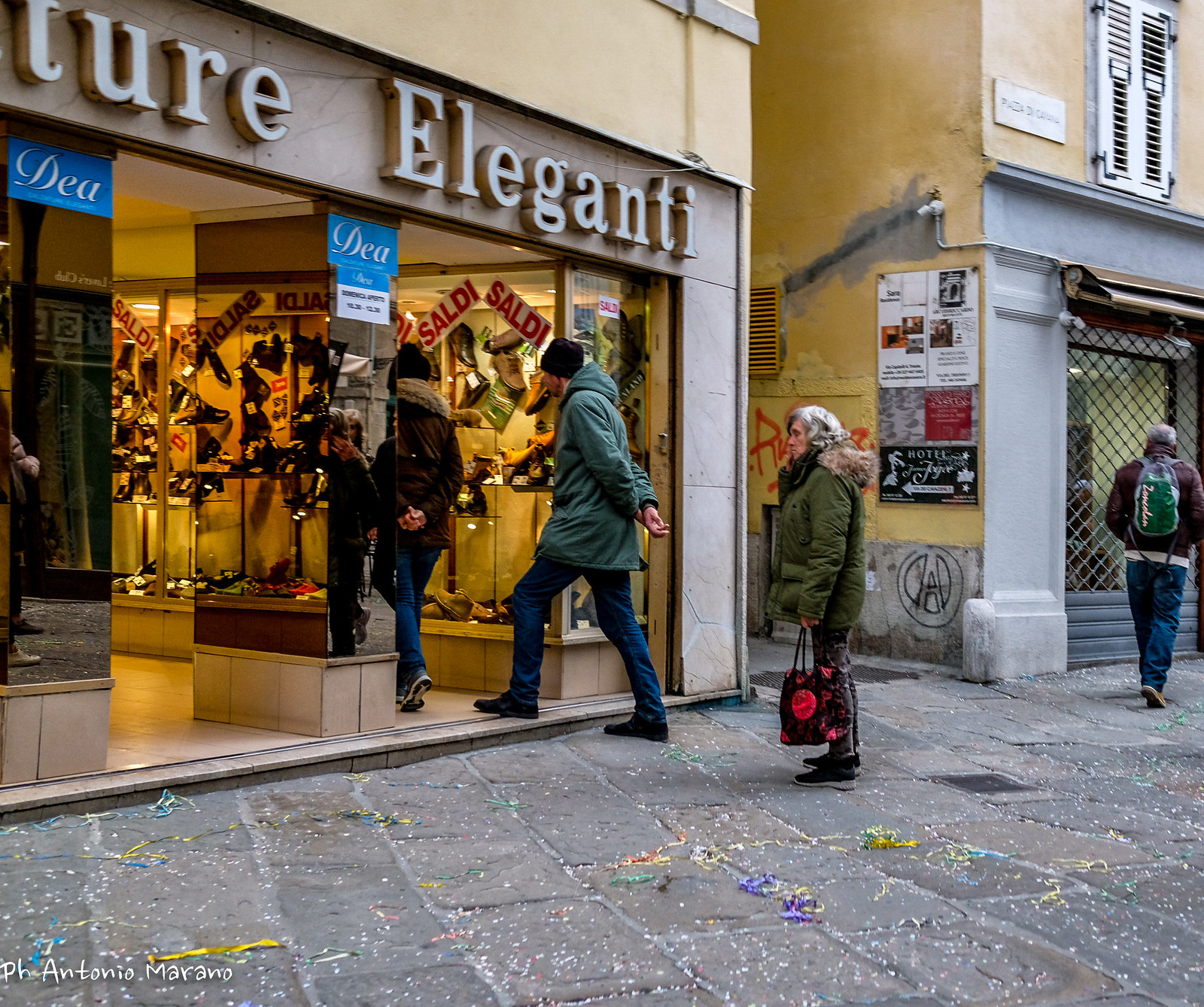In this image, there is a bustling street scene set outdoors in the middle of the day, likely downtown. The ground surface is a wide stone brick walkway in shades of gray. The scene is centered around a storefront with its wide-open doors, displaying the word "elegante" in white letters on a gold-colored wall. A window display with a goldish hue showcases what appears to be shoes, adding a touch of sophistication to the store's façade. 

Three individuals, dressed in coats suggesting chilly weather, stand directly in front of the store, centrally positioned in the image. To the top left of the image is another building, which appears to be part of the same storefront or a neighboring shop. The upper right corner of the image features a cut-off structure, making its purpose unclear, but it’s adjacent to the primary storefront.

The colors in this image range from gray to light blue, white, yellow, blue, purple, red, pink, yellow, and green, enhancing the urban atmosphere. Notably, there is another yellowish building next to the storefront with a gray façade, partially fenced and adorned with graffiti, adding an eclectic vibe to the scene. There is no readable text other than the elegant store inscription, suggesting the text might be in a different language.

Overall, the image captures a dynamic moment in a downtown shopping district with diverse architectural elements and a lively pedestrian presence.